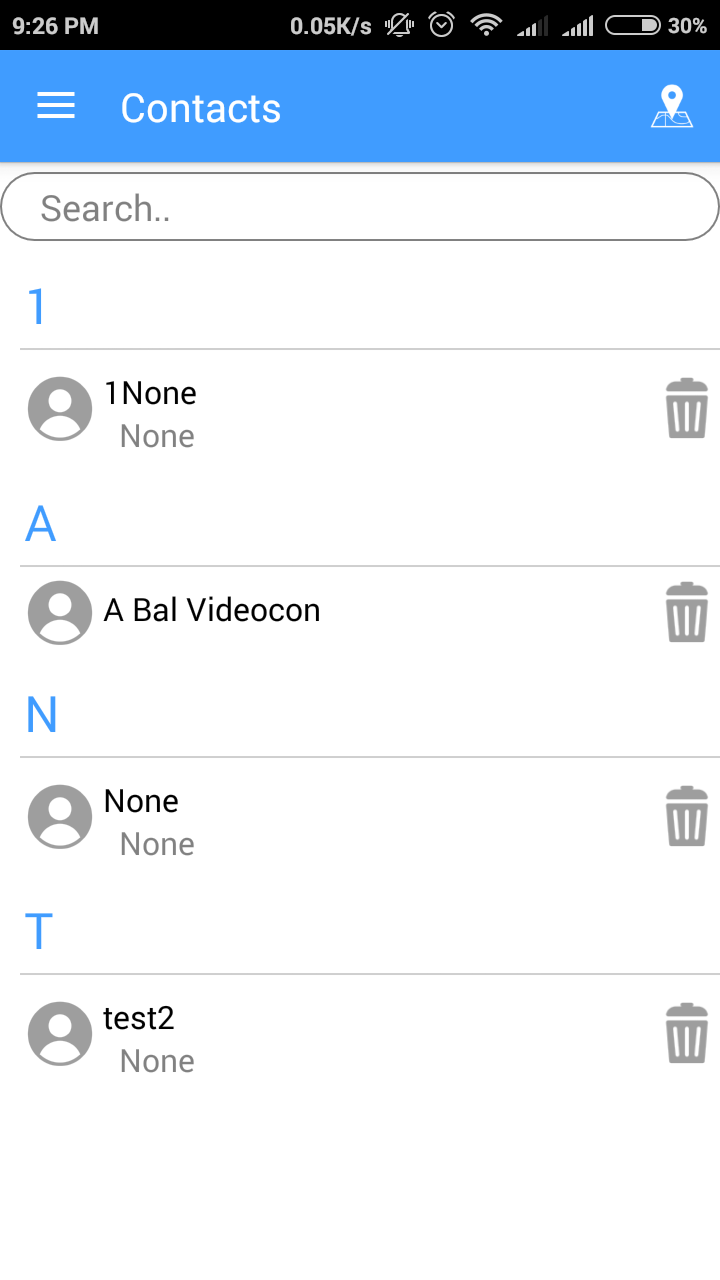The image is a screenshot taken from a mobile device that displays a contacts application. The screen has a white background. At the top, there is a black horizontal status bar. On the left side of this bar, the time is displayed as 9:26 p.m., while the right side features various icons including a battery icon indicating a 30% charge.

Beneath the status bar is a blue navigation bar with the word "Contacts" written in white text. Directly below this is a search window, with the word "Search" appearing in gray within the input field.

The main portion of the screen displays contact entries organized in rows. There are a total of four contact rows. Each row includes contact information on the left side and a delete icon on the right side. The delete icon, which is partially visible, is likely a trash can symbol, commonly used for deletion functions.